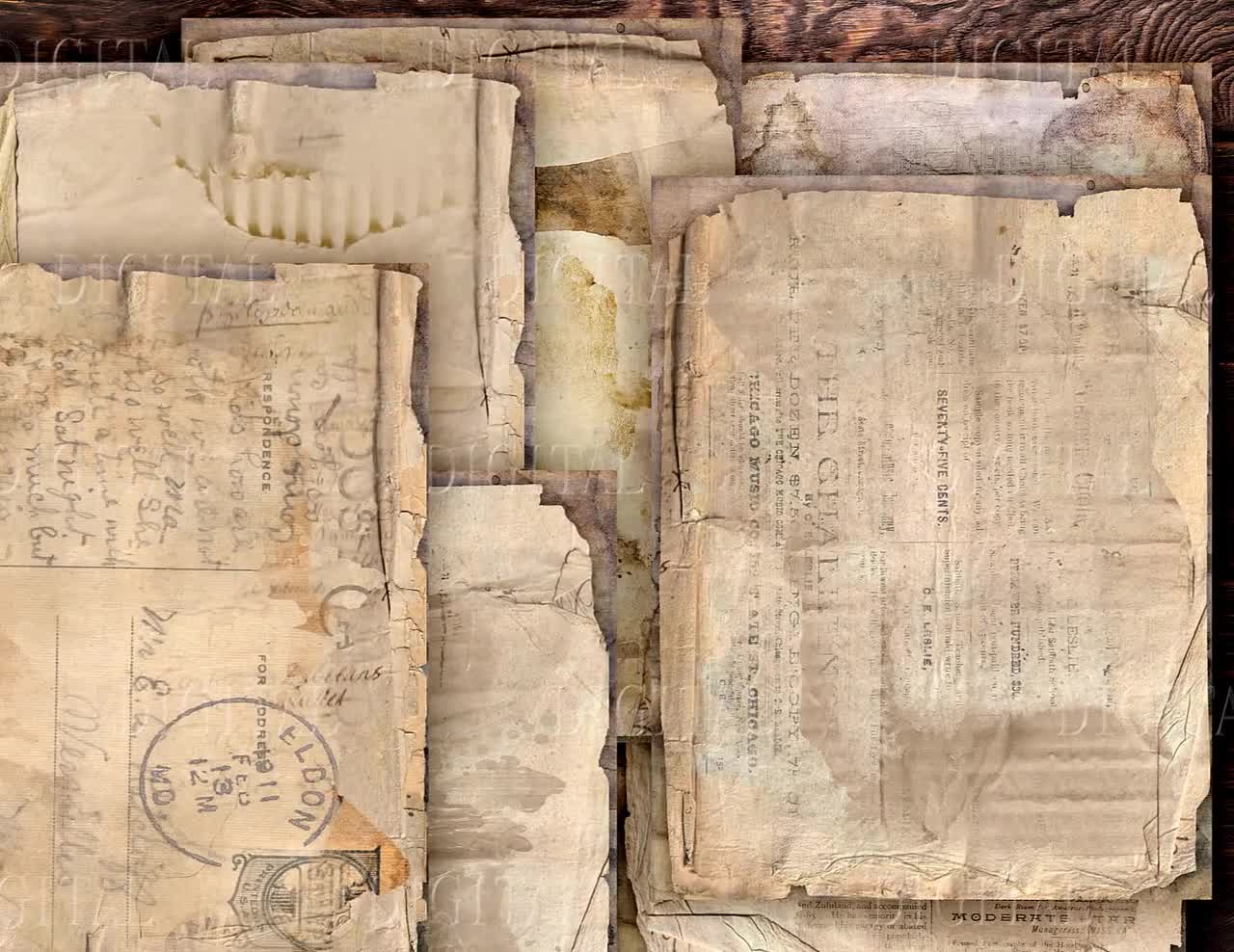This is a color photograph in a rectangular, landscape orientation, measuring approximately 6 inches wide by 4 inches high. The image features a collection of well-worn and weathered postcards and papers, some of which are stacked. These aged documents exhibit significant damage, including water stains, faded ink, and tattered edges. The most discernible postcard features a faint postmark from Eldon, Maryland, and potentially dates back to 1911 or 1913, though the exact date is unclear due to the wear.

The documents in the photograph appear in various states of decay: some are so deteriorated that the text is nearly illegible, while others have partially discernible print, such as a center stamp indicating "75 cents." Among these items, one stands out as severely damaged, showing only the corrugated layer of the cardboard. 

The background of the scene is a dark brown wooden table, partially obscured by the papers, with visible thick, round wood grain patterns. An item on the right side of the image, possibly a newsletter, is turned on its side with some visible gray type. The entire photograph bears a watermark of the word "digital" repeated multiple times in a transparent bubble effect, indicating that it may be a piece of digital artwork mimicking vintage print items.